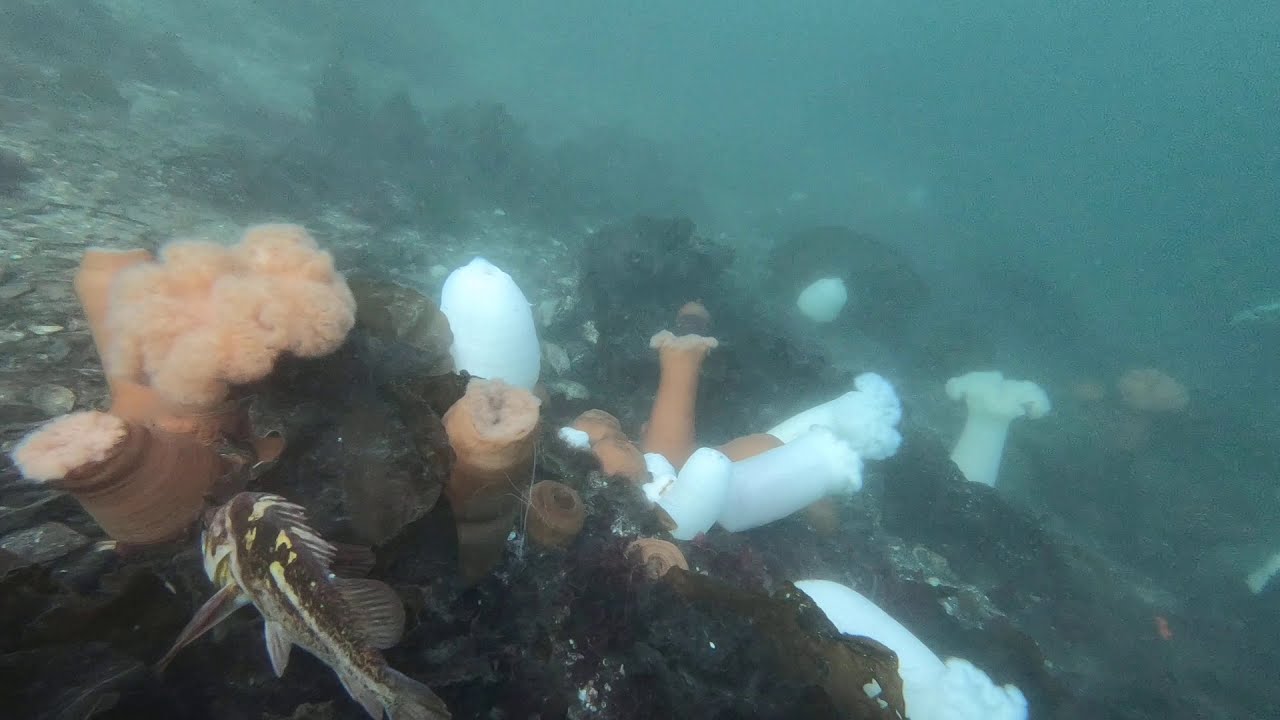The underwater scene is drenched in a blue tint, typical of murky water. The view reveals an ocean floor peppered with a variety of rocks in hues of black and tan, interspersed with occasional patches of gray dirt where no fauna thrives. Multiple sea plants, appearing fluffy and mushroom-like, grow from the rocks; these are mostly white and light orange, suggesting some form of marine fungus or sea mushrooms.

In the bottom left corner, a distinct triangular-shaped fish with long fins catches the eye. It is predominantly tan adorned with yellow spots and white lines, hinting at a possible grouper. The top right of the image fades into a murky blue, shrouded in low light that limits visibility and adds to the mysterious ambiance of the underwater scene.